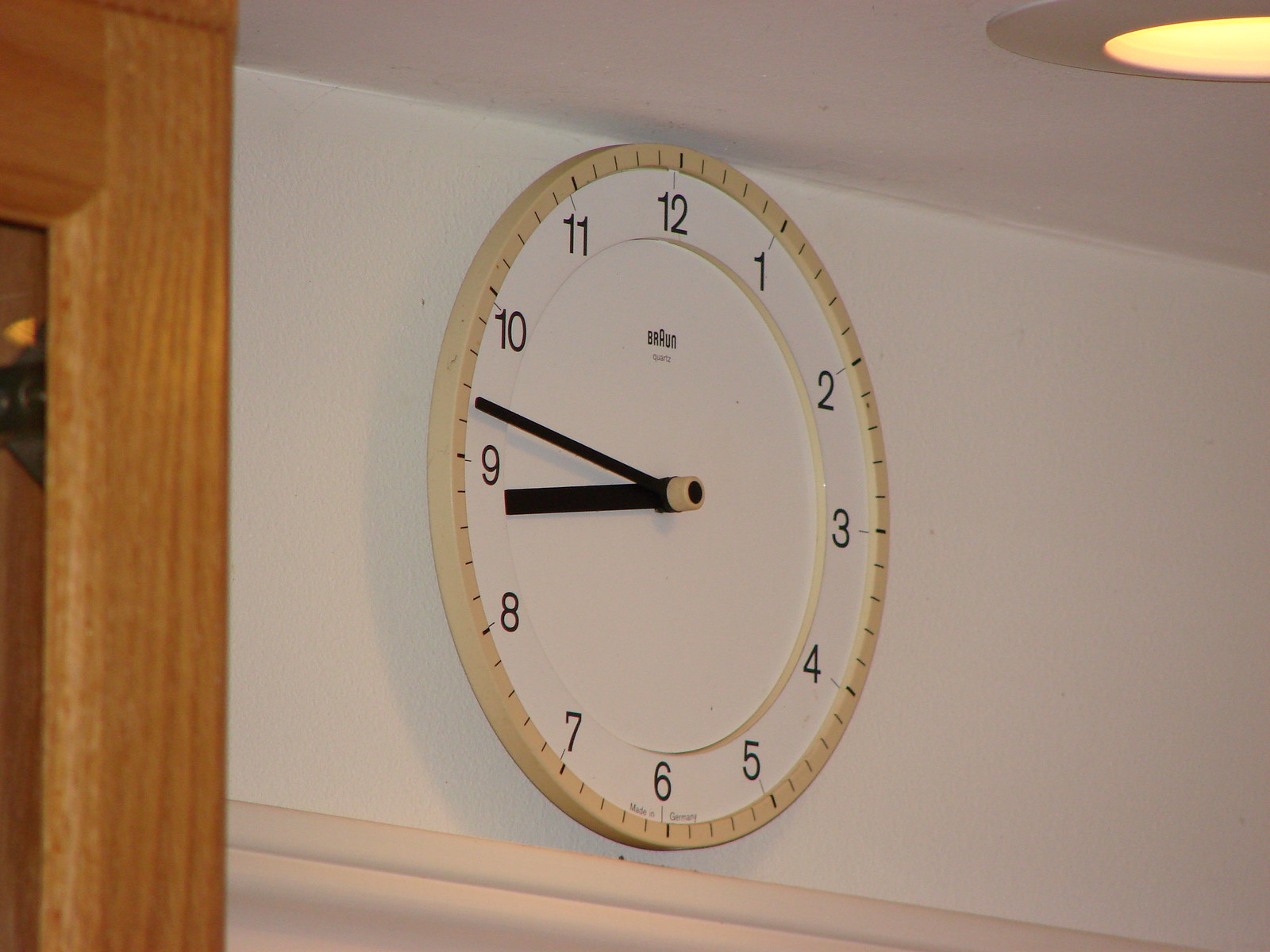The photograph captures a round wall clock with a beige rim hanging almost at ceiling height on a white wall, positioned slightly above a doorway. The wall and ceiling are painted white, and there is a light wood doorframe visible on the left with white wainscoting running across the wall. A recessed light fixture is observed in the upper right corner of the ceiling. The clock face is typical white, featuring black numbers and black minute and hour hands, with the minute hand between the 9 and 10, and the hour hand nearing the 9, indicating the time is approximately 8:47. The brand name "Braun" with a larger "A" is printed below the 12, along with the word "Quartz," while the phrase "Made in Germany" is found near the 6.